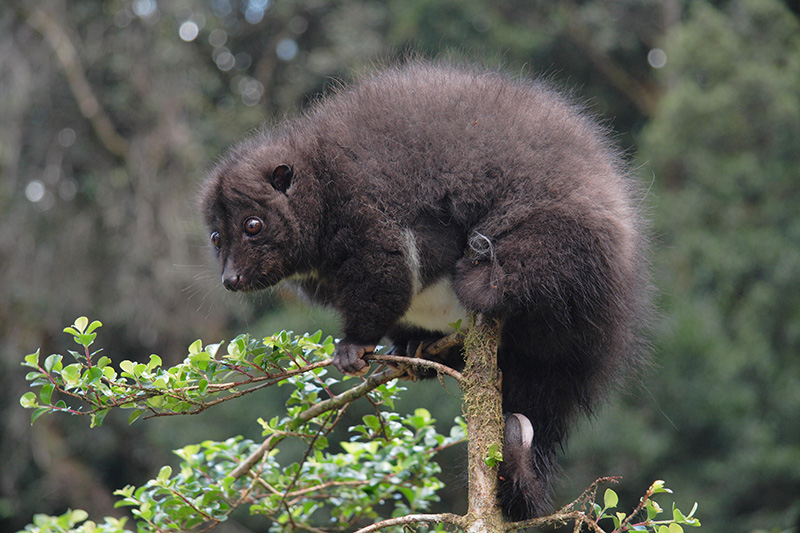The photograph, sized approximately two inches high by three inches wide, captures a small, fuzzy, brown animal perched on the top of a light brown tree, against a background of blurred green foliage and brown branches. The creature, reminiscent of a monkey or similar small mammal, has dark brown fur that grows darker towards its lower body and features a furry tail draped down the tree. The animal’s face is turned to the left of the image, showcasing a pointy brown nose, small brown ears positioned towards the top side of its head, and big, round, beady brown eyes. The branch it clings to is adorned with shiny, green and yellow leaves, suggesting it might feed on these leaves. Despite its small head and tiny ears, the animal has a notably fuzzy body, estimated to weigh between eight to twelve pounds. The overall setting appears to be a wooded area, captured in broad daylight, adding a natural, serene ambiance to the scene.